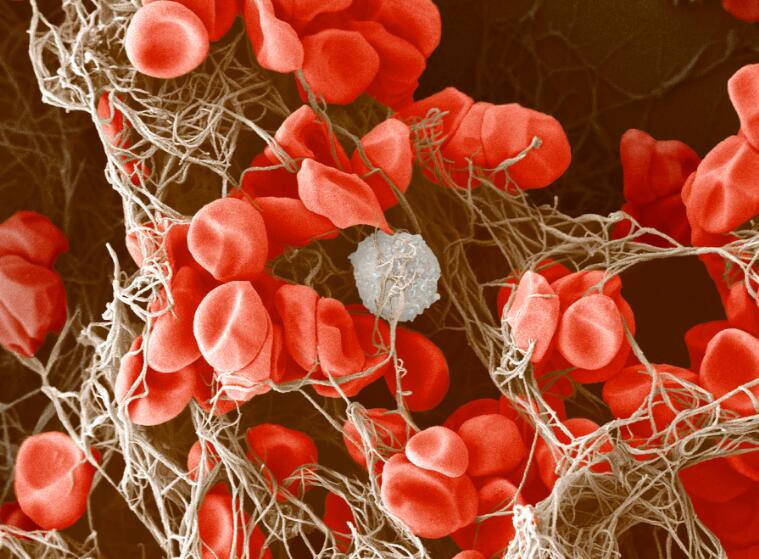The image depicts a highly artistic and possibly magnified or digital representation featuring an intricate dance of light-brown twine or twig-like structures interwoven among multiple elongated and slightly indented red, rose petal-like shapes with subtle white highlights. These shapes, clustered predominantly in the upper left, cascade diagonally downwards to the right, creating a dynamic yet delicate web-like arrangement. At the very center of this subdued and unsaturated scene lies a perfectly round, crystallized globule resembling an ice ball or a piece of hail, adding a focal point that anchors the composition. The overall image exudes a blend of organic and synthetic elements, resulting in a visually engaging and meticulously designed artwork.